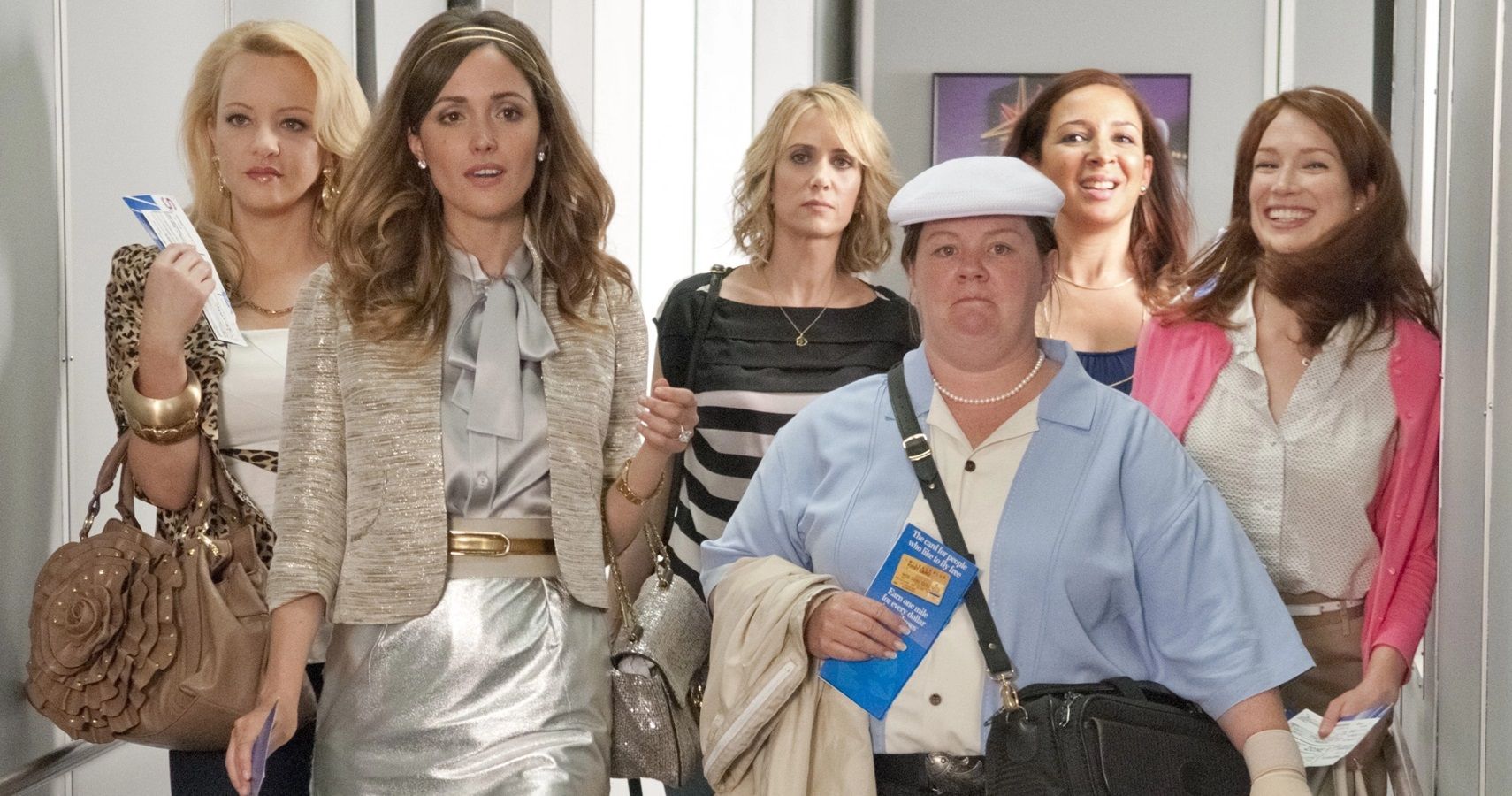This color photograph, a still from the movie "Bridesmaids," captures six distinct women standing in what appears to be a white office or hallway with panel curtains. The woman on the far left, with determined blonde hair, clutches a piece of mail or a plane ticket while sporting a brown purse and gold bangle. Adjacent to her is a woman styled in a metallic silver ensemble, walking casually with long hair and a confident demeanor.

In the background, there’s a shorter woman with striking short blonde hair wearing a striped boat neck top, and beside her, another woman with a disgruntled expression donning a pearl necklace, white cabbie hat, and a men’s style pale blue shirt with a white stripe. She has a black shoulder bag.

Behind the frustrated woman is a smiling dark-haired woman, barely visible except for a patch of blue around her neckline and a gold necklace. To her right, standing prominently, is another smiling brunette with long hair, clad in a white button-down blouse and a pink cardigan while holding a piece of paper, possibly a plane ticket.

In this scene, each character’s unique personality and attire are highlighted, from the determined blonde with a leather flower motif purse to the classy silver-clad woman with a headband and earrings, reflecting a blend of determination, elegance, and casual styles.